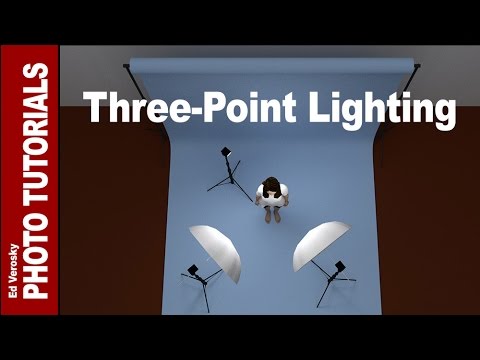This image is a detailed 3D rendering used as a tutorial for photographers about three-point lighting setups. The scene features a woman with long black hair and a white shirt standing on a photographic set viewed from above. The backdrop is a light blue paper that extends onto the floor, creating a seamless background. There are three black tripods with lights arranged around her: one to her left and one to her right, each equipped with white diffusing umbrellas, and one more behind and to her left without an umbrella. The lighting setup provides a classic three-point lighting arrangement, illustrating the correct positioning for a photo shoot. The composition is framed by a red vertical bar on the left side with white text that reads "Ed Verosky Photo Tutorials" and black bars at the top and bottom. Centered at the top of the image is the title "3-Point Lighting" in white text.